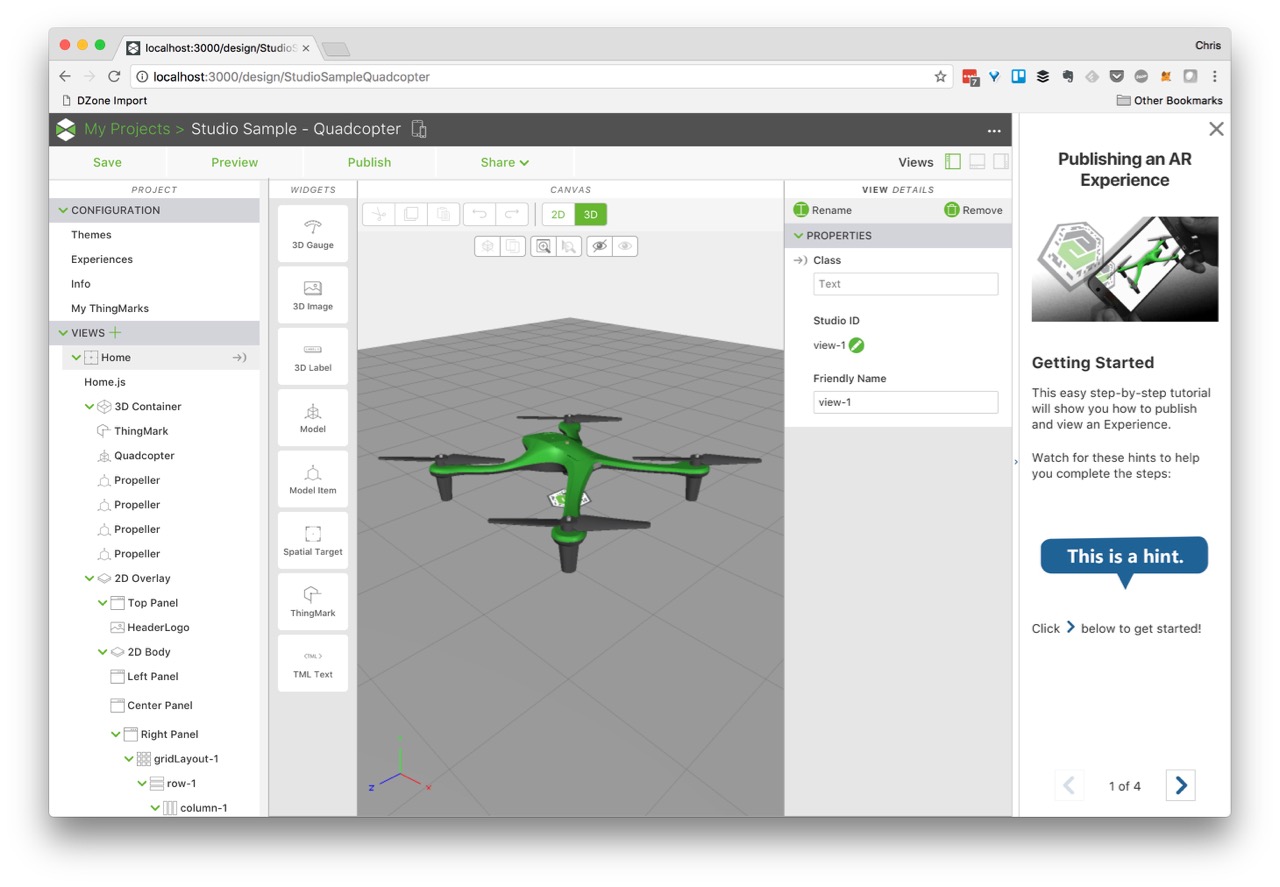Screenshot of a software interface showing the programming of a bright green quadcopter. The quadcopter, equipped with four propellers, is positioned on a gray checkered floor within the design canvas. The top of the interface displays a tab labeled with the URL "localhost:3000/design/studio," truncated at the end. The sidebar features two expanded drop-down sections: "Configuration" and "Views." 

Within "Configuration," the options listed are "themes, experiences, info, my thing marks." The "Views" section is more extensive, structured like a nested tree, containing:
- home
- home.js
- 3d container
- thing mark
- quadcopter
- propeller (repeated 4 times)
- 2d overlay
- top panel
- header logo
- 2d body part
- left panel
- center panel
- right panel
- grid layout (with sub-items: one row, one column, one)

The interface is populated with various 3D widgets and buttons such as "3d gauge, 3d image, 3d label, a model, model items, spatial target, thing mark, and TML test."

On the right side, there are additional sections for "views" including options to "rename" or "remove." It also shows properties and classes labeled as:
- text
- studio ID: view 1
- friendly name: view-1

An instructional panel titled "Publishing an AR experience" guides users through the process, offering a step-by-step tutorial. This panel includes hints within blue speech bubbles, directing to "click > to get started," with pagination indicating "1 of 4." The left arrow is grayed out, and the right arrow is interactive.